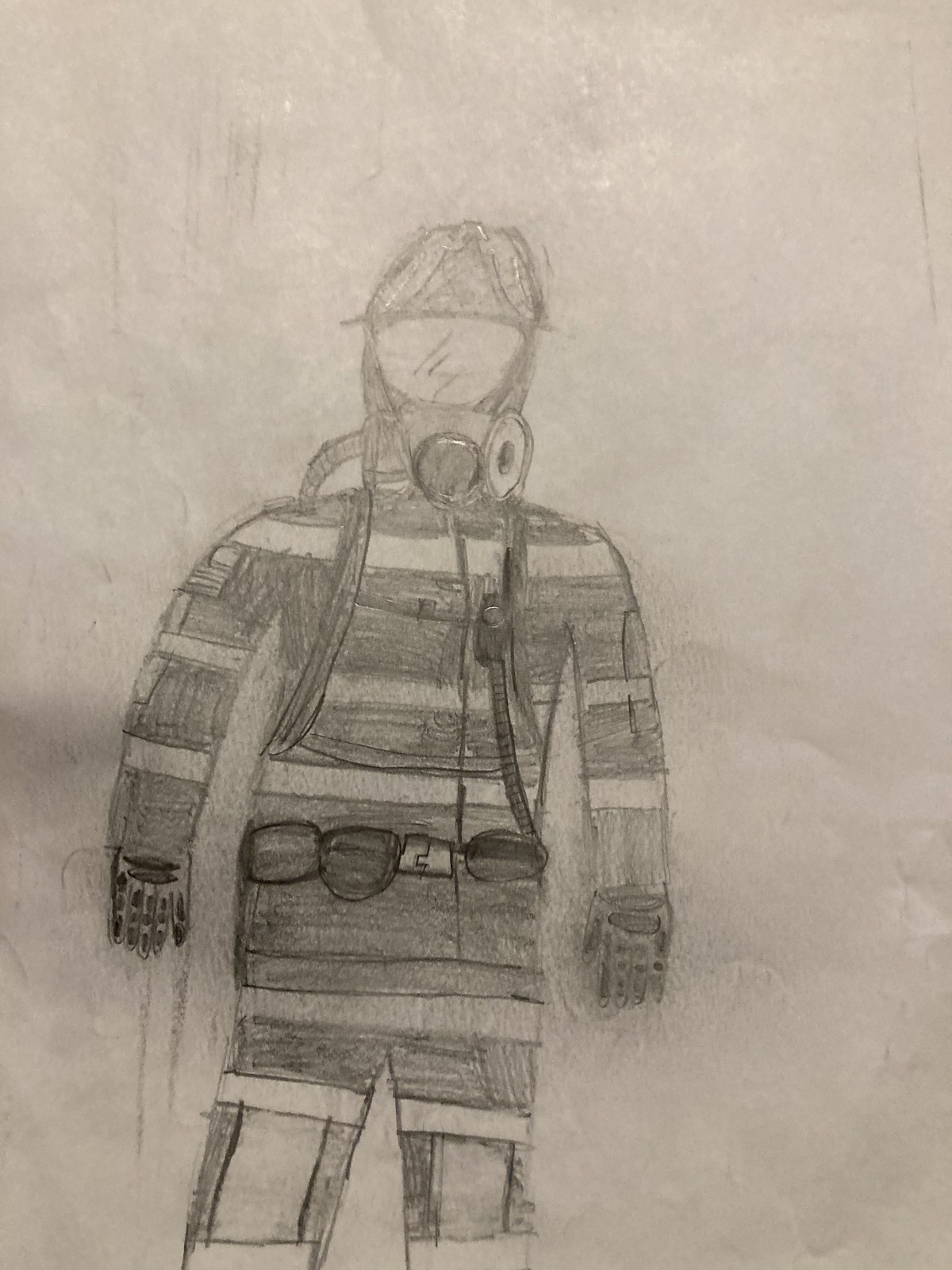The image depicts a detailed pencil drawing of a firefighter set against a textured, grayish-white background of rough paper. The firefighter is fully equipped and depicted from head to toe. They are wearing a helmet with a visor and a gas mask, which conceals their eyes. Their attire includes a vest adorned with horizontal white stripes, a belt with multiple pouches, and pants featuring several horizontal and vertical white rectangles. The torso and the harness around the belt are colored in darker shades. The drawing fills most of the paper, extending from near the bottom to about 20% from the top.